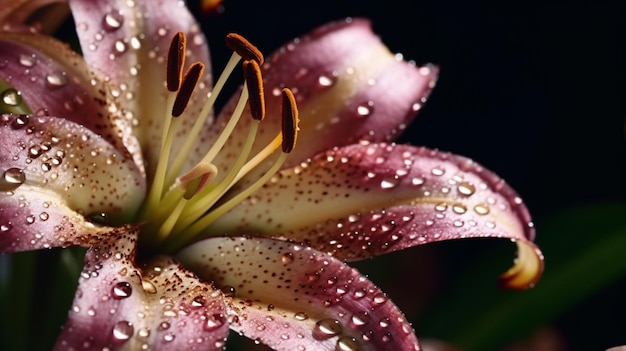The close-up image showcases a stunning tiger lily flower with delicate purple petals that curl gracefully at the tips. Each petal is adorned with tiny, bead-like droplets of water, highlighting the flower's intricate beauty. The flower, positioned towards the left of the frame, displays a striking gradient from creamy beige at the center to rich magenta and maroon at the ends, which are pointed and curled. The petals' interior features subtle hints of yellow and speckled maroon markings, adding depth and texture. Long, slender filaments with small, fuzzy seed parts, cream-colored to brown at the tips, emerge from the flower's core, where pollen is visibly settled. The background is predominantly black, creating a stark contrast that enhances the vivid colors and delicate details of the lily, with a hint of greenish shade suggesting the presence of a leaf at the lower right.